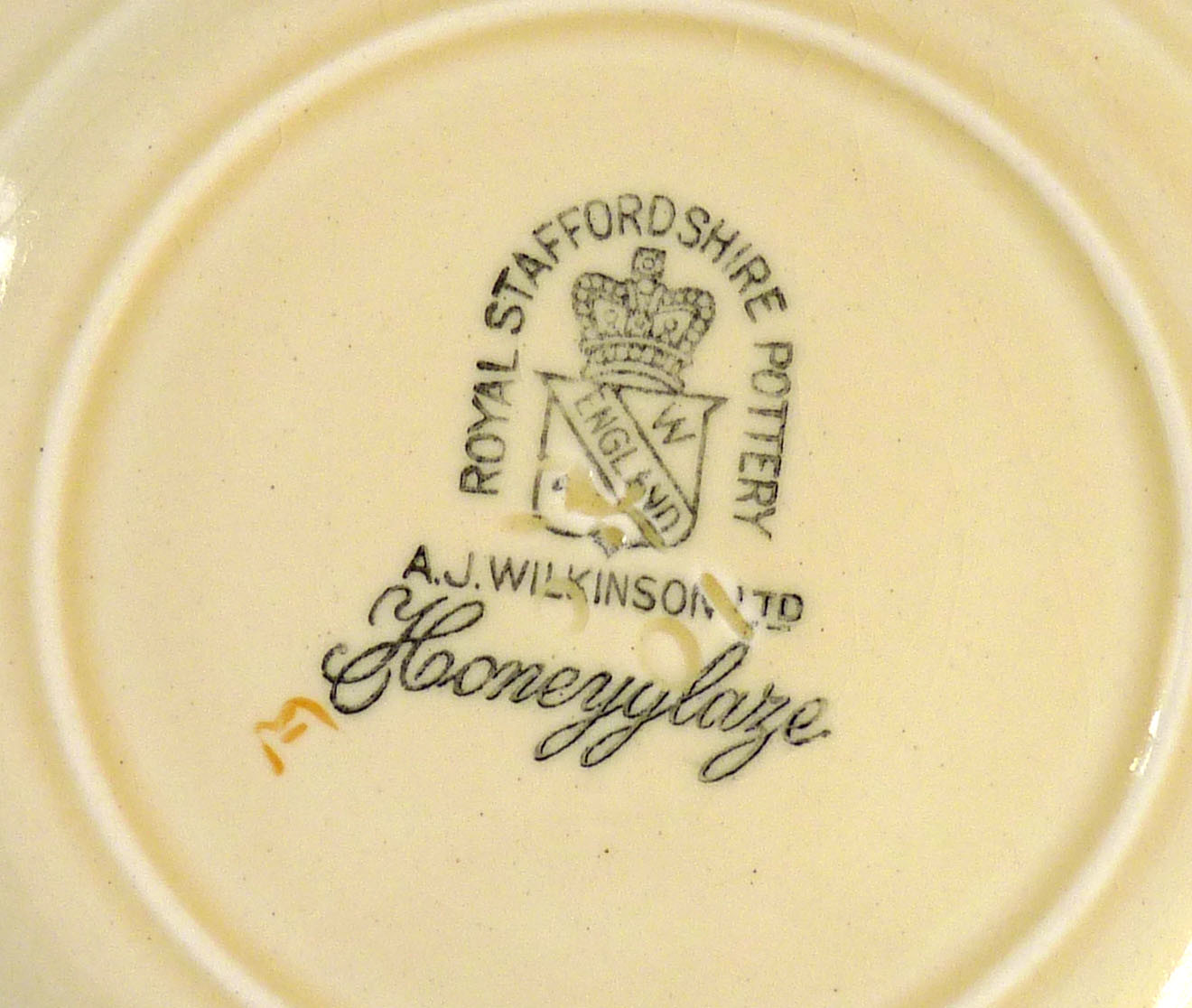This landscape-oriented photograph showcases the underside of a ceramic plate, predominantly cream in color with black lettering. The focus is on a detailed black stamp identifying the plate's provenance. At the center of the stamp is a logo featuring a crown atop a shield, under which the word "England" is inscribed in a sash. Encircling this logo in an inverted U-shape, the lettering reads "Royal Staffordshire Pottery." Below this, the text "A.J. Wilkinson Ltd" is clearly marked, followed by the cursive writing "Honey Glaze." Adding a touch of charm, a small yellow bee is sketched near the cursive text. There are also some cream-colored, slightly raised edges on the bottom of the plate and faint printing that appears to read "1-0", blending into the plate's surface. The intricate detailing of the stamp and the soft cream tones highlight the craftsmanship of this piece of ceramics.